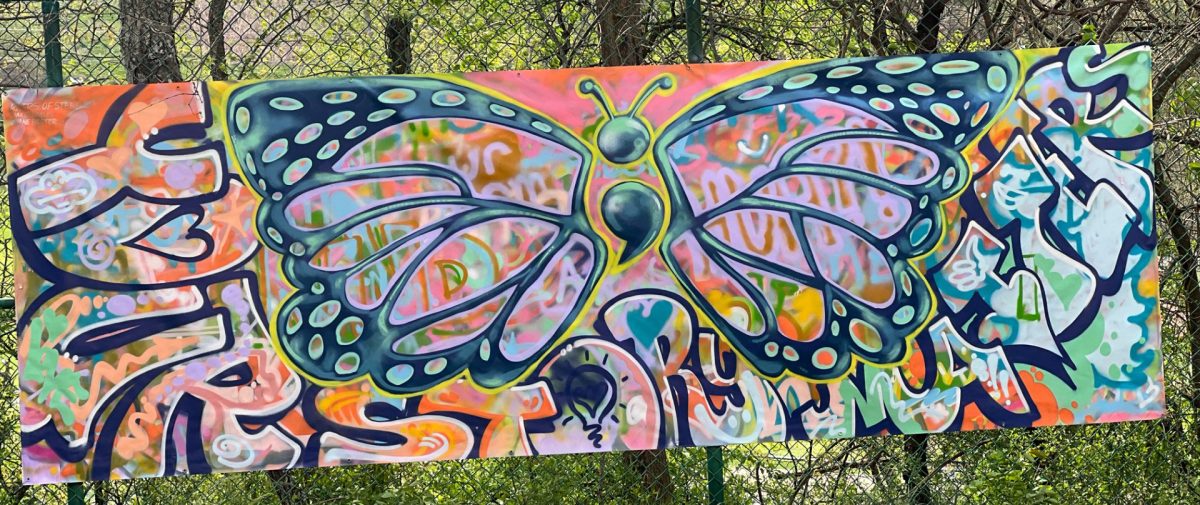The image features a vibrant, graffiti-styled banner hanging on a chain-link fence, with the fence positioned in front of a lush, green area filled with trees and foliage. The banner, roughly three times as long as it is tall, showcases a large, colorful butterfly at its center. This butterfly has a unique design with a blue circular body, curvy antennae, and wings that reveal the background through transparent sections. The wings are primarily blue and adorned with circle patterns. The background of the banner is a mix of bright, tie-dye-like colors, predominantly orangey-pink. White, bubble-like text encircles the butterfly, reading "Your story matters." The scene is set outdoors during the daytime, and the fence includes green metal poles, blending into the natural surroundings.